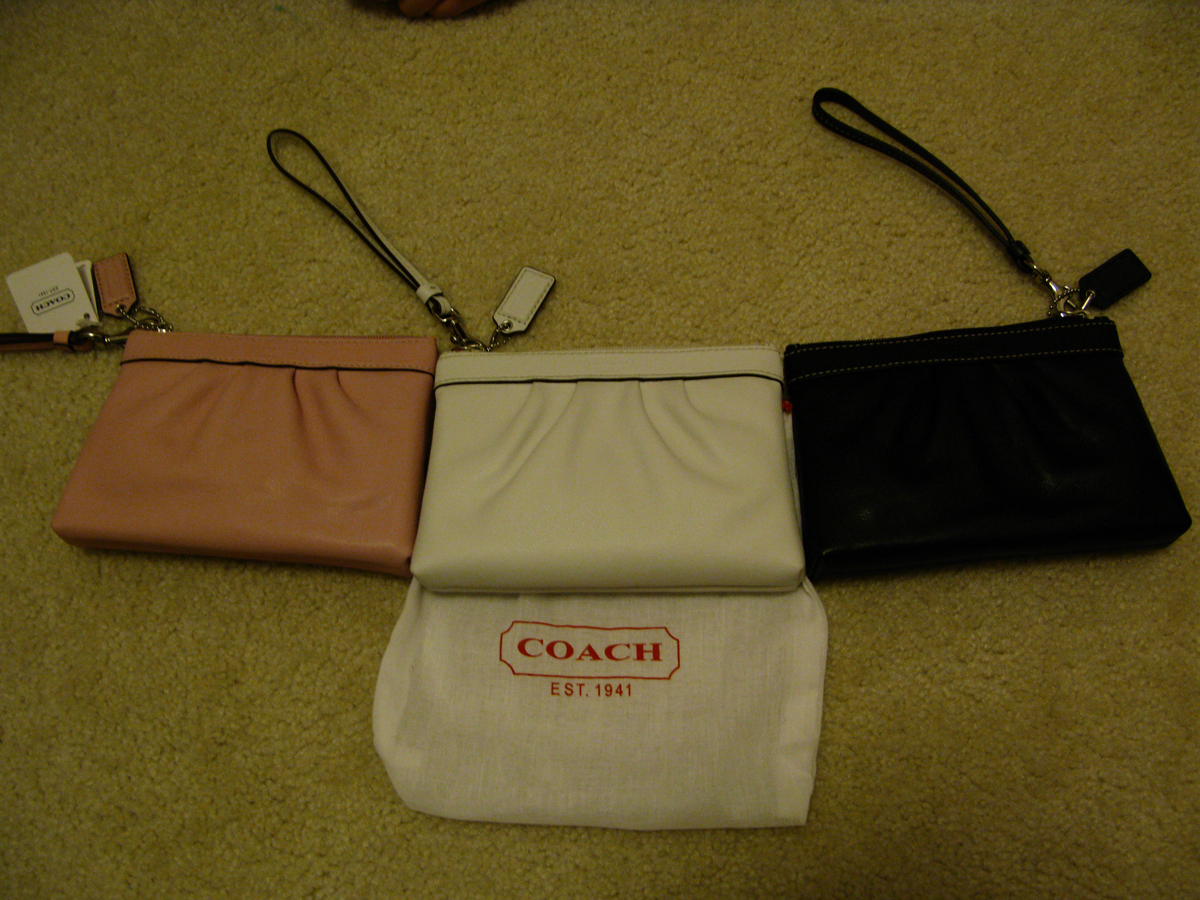The photograph features three small Coach handbags, neatly aligned in the center of the image. Each bag is distinct in color but shares the same shape and size. The handbag on the left is a light pinkish cream color and includes a keychain made of the same material, along with a Coach tag on the top left corner. The center bag is white with a piece of white vinyl material below it, showcasing the Coach logo and "Established 1941." The right-hand bag is black, possibly made of suede, and appears to be another Coach bag. All three handbags have their original tags attached and their straps are visible above them. They are laid out on a clean, beige cream shaggy carpet, which serves as the subtle background for the main focus of the image.